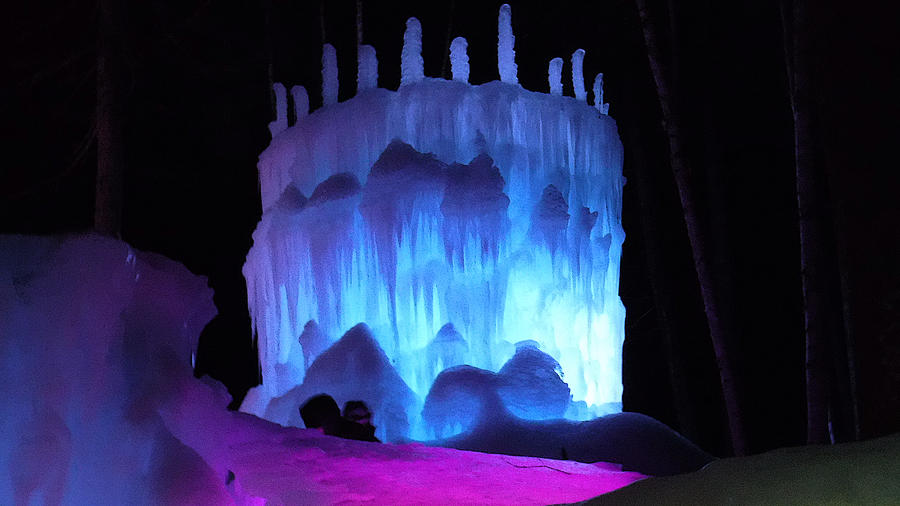This image captures a vast and intricate outdoor ice sculpture that evokes a majestic ice castle, reminiscent of something from the movie "Frozen." The sculpture features towering turrets and a ridge with embedded, cave-like details such as stalactites. Illuminated from within, the sculpture glows with enchanting hues of blue, purple, and pink, creating an ethereal ambiance against the dark backdrop dotted with indistinct trees. Scattered around the base of the sculpture are intriguing shapes that resemble balls or faces, adding to the magical scene. In the foreground, possibly captured by someone standing on a nearby road, are the faint outlines of what might be a father and his daughter, gazing in awe at the marvel before them. Another smaller ice sculpture with pink and purple lighting stands to the left, while a faintly green hill appears to the lower right, completing this captivating winter wonderland.